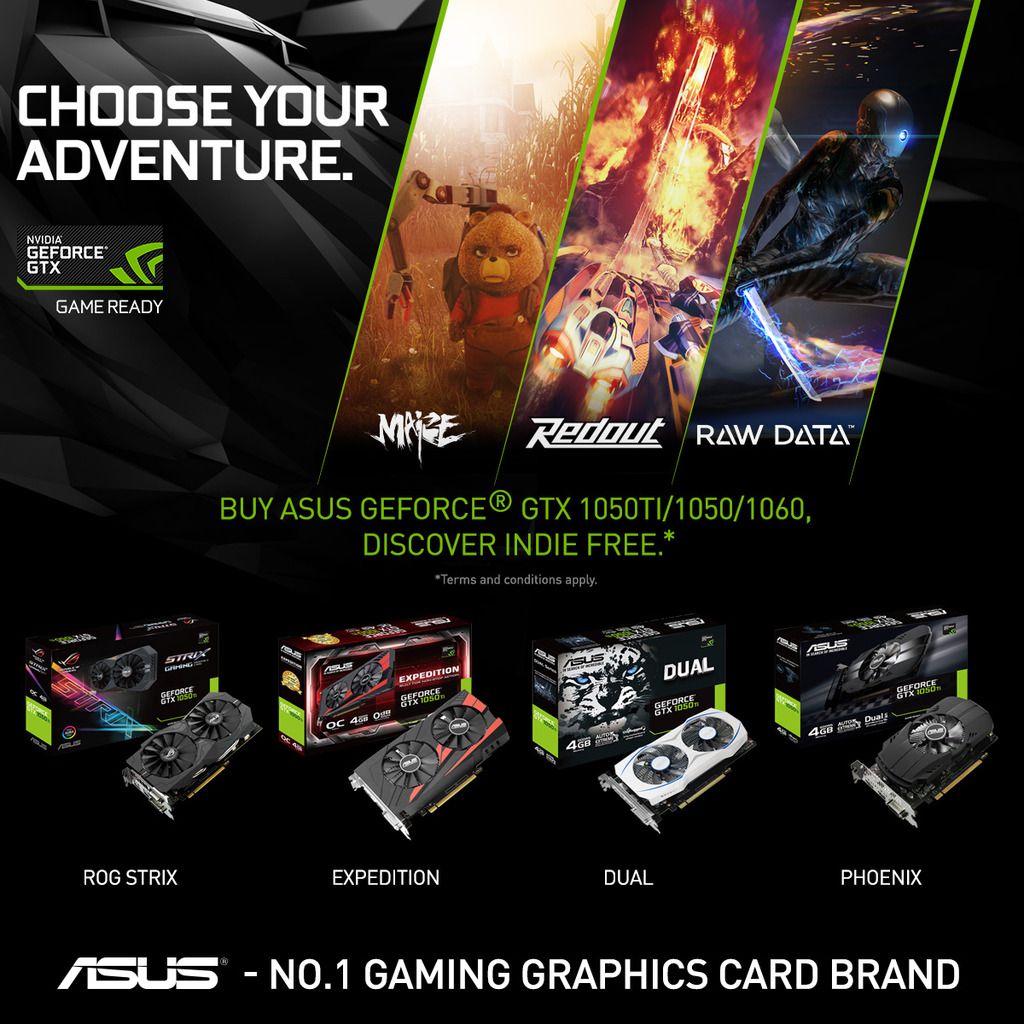This image is a screenshot from a website with a predominantly black background. At the top, there are graphics featuring thick, dimensional gray lines. Overlaid text in all capital letters reads "CHOOSE YOUR ADVENTURE." Below, three distinct panels are separated by a horizontal lime green line. 

In the center, a series of concentric circles progressively increase in size downwards. The text "Photobucket" appears prominently in this section. Nearby, additional text reads "by ASUS GeForce GTX 1050 Ti / 1050 / 1060" in lime green. This is followed by the bold text "DISCOVER INDIE FREE."

A white banner emerges, stating "Protect more of your memories for less." Below this, branding graphics include "ROG Strix," "Expedition," "Dual," and "Phoenix."

At the bottom of the image, the text "ASUS" is followed by a dash and the words "No. 1 Gaming Graphics Card Brand." The "No." is abbreviated and followed by a space before the numeral one. Overall, the image features a blend of promotional and branding elements with a bold design and striking lime green accents on a dark background.